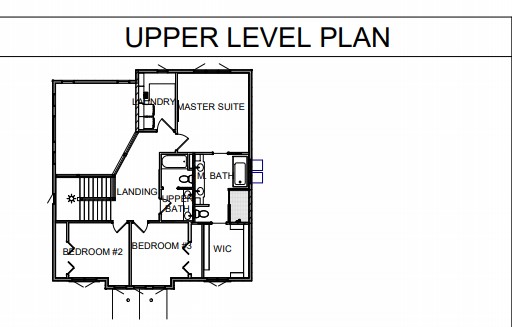The image depicts a detailed upper-level floor plan on a white background. At the top of the image, in bold, black, capitalized text, it reads "UPPER LEVEL PLAN" between two thin horizontal black lines. Additionally, there is a vertical black line along the right edge of the image.

The floor plan itself is a square layout with labeled compartments. Starting from the top left, there is a designated "Laundry" area featuring a washer and dryer. Adjacent to this is the "Master Suite," which appears spacious and leads into a connected bathroom. The bathroom, detailed with fixtures such as a toilet and vanity, extends to an area labeled "Upper Bath."

The floor plan also includes a "Landing" area, and moving further to the right, it highlights "Bedroom 2," positioned beside "Bedroom 3." Notably, "Bedroom 3" features a small extension labeled "WIC," indicating a walk-in closet.

Overall, the image is a clear and concise representation of the upper level's layout, providing a comprehensive view of each designated room and area.